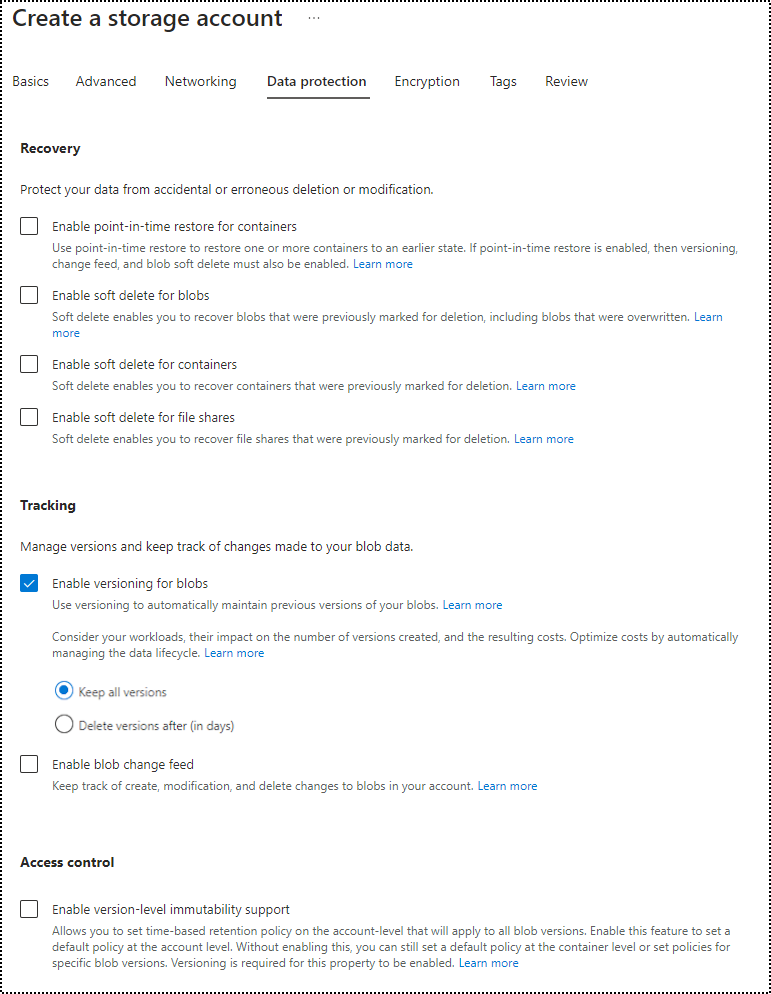The image is a screenshot of an online application with a clean, white background. The primary function displayed is "Create a Storage Account," prominently located in the upper left corner. Below this title, there's a horizontal menu bar showcasing various tabs: "Basics," "Advanced," "Networking," "Data Protection," "Encryption," "Tags," and "Review." The tab "Data Protection" is underlined, indicating it's the current selection.

On the left side, in black text, the word "Recovery" is visible. Underneath "Recovery," a message reads: "Protect your data from accidental or erroneous deletion or modification." Below this message, there are four empty checkboxes, each with instructions listed to their right. Furthermore, beneath these checkboxes, the word "Tracking" is written in black. The screen is primarily focused on options related to data protection and recovery within the application.